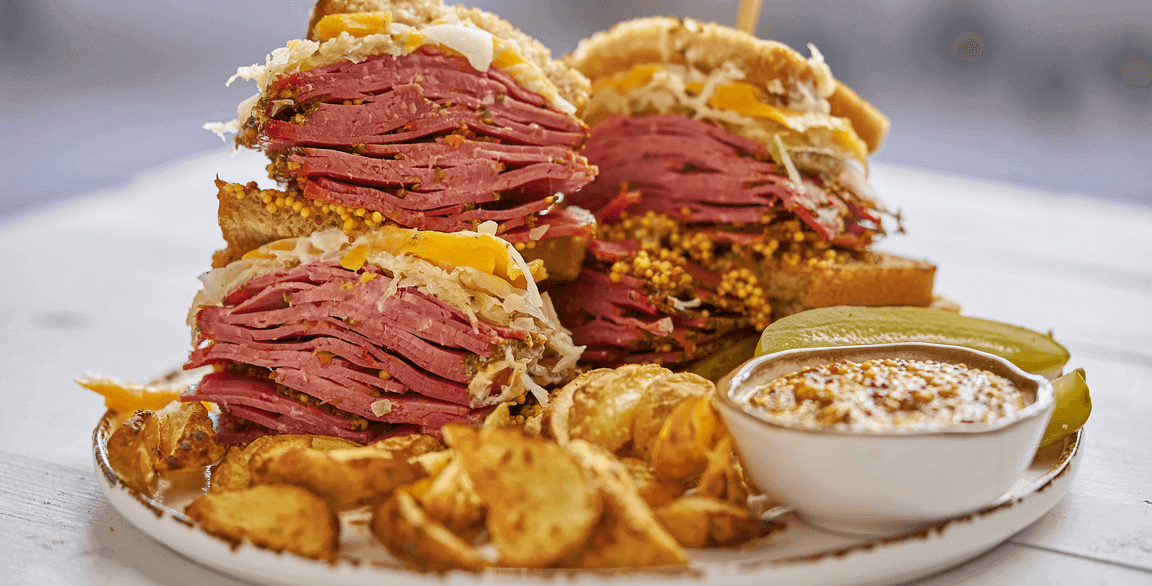This horizontal rectangular image features a large plate of hearty food, suitable for multiple people. The focal point is a collection of substantial sandwiches, each cut in half to reveal generous fillings of at least two inches thick, suggesting a meat such as ham, corned beef, pastrami, or roast beef. These sandwiches appear to be Reuben sandwiches, as they are likely filled with meat, cheese, and sauerkraut. Piled high at the back, the sandwiches are accompanied by thick potato wedges or slices, front and center. To the side, there's a bowl potentially containing mustard or a dip, suitable for both the sandwiches and the potatoes. Peeking from behind the dip bowl are several pickles, adding to the variety of this meal. Overall, this image showcases an appetizing array of meat-heavy sandwiches, crispy potatoes, tangy pickles, and flavorful dips, representing a hearty and satisfying lunch.